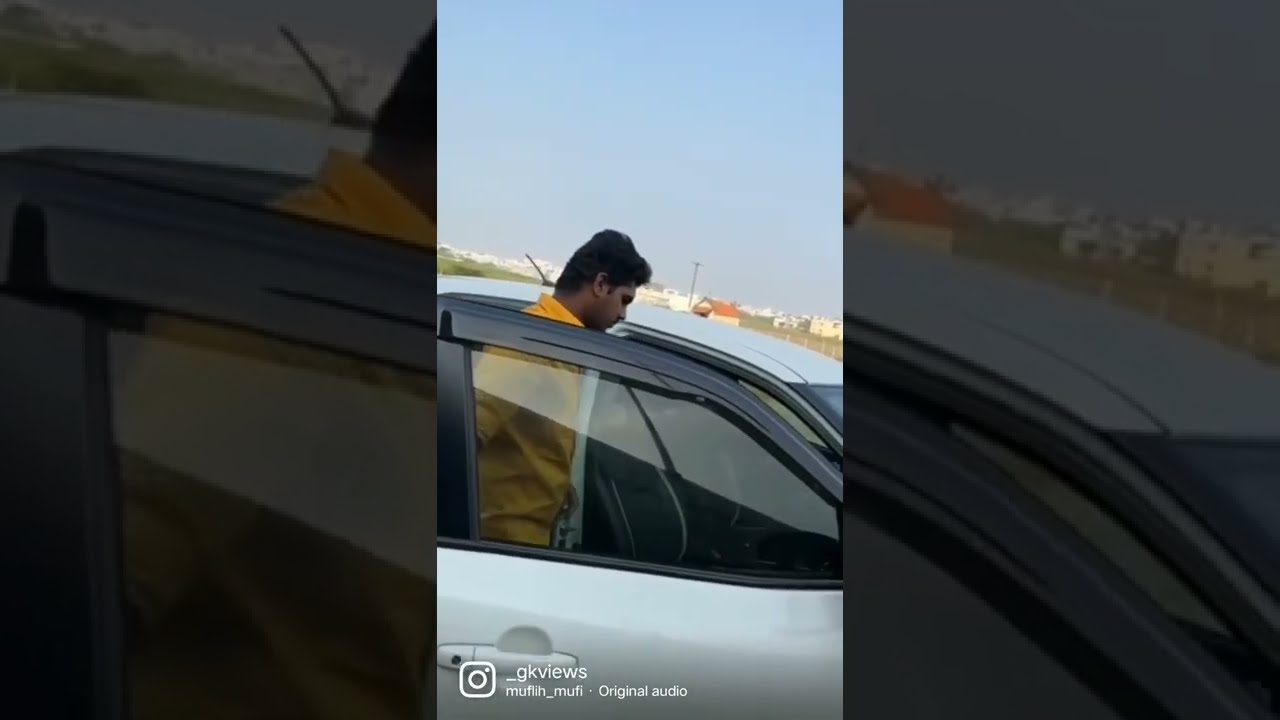The image is a three-panel composition, with a central focus panel that is brightened and two flanking panels on the right and left that are translucent and darkened, offering close-up views from different angles. At the center of the image, a silver car with black-framed windows and rain protectors on the door is depicted. The car’s passenger door is ajar, revealing a man wearing a long-sleeve yellow shirt. This man, who has black hair and dark brown skin, is either entering or exiting the car, with his head tilted downward, looking inside. The car features black leather seats with white piping, and a small black antenna is visible on the roof.

The background scene visible through the car’s windows and above the doorframe includes the horizon, a skyline with various structures, and some greenery, particularly on the left side. These elements are more pronounced in the flanking panels. The right panel shows the town in the background, part of the skyline, and the front section of the car door. The left panel highlights the back portion of the door, the man’s torso, neck, and antenna, along with snippets of trees and buildings.

An Instagram logo appears beneath the main image, along with text that reads "OK views" or "GK views."